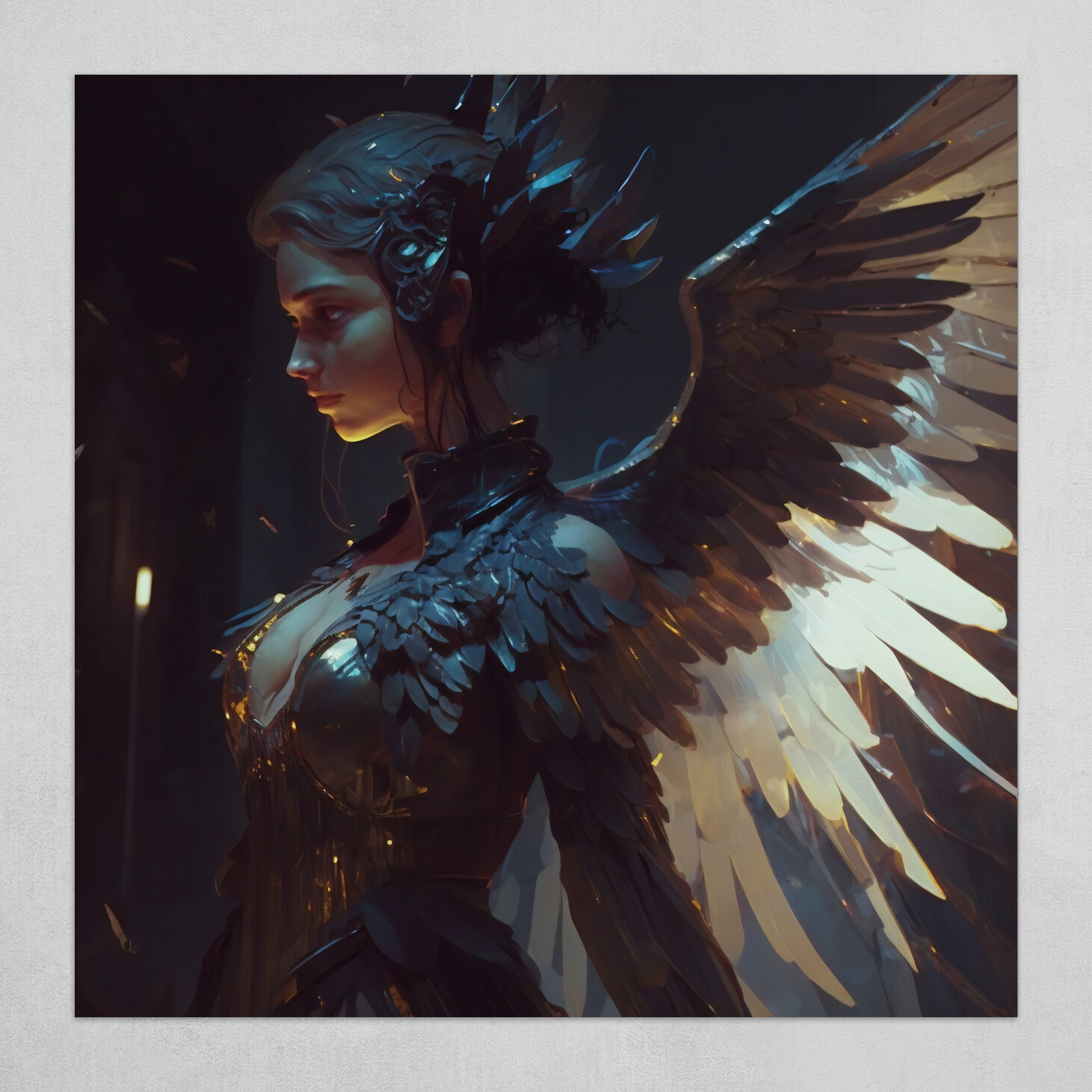The image depicts an intricately illustrated woman with wings, seemingly generated by AI. She is positioned slightly to the side, directing her gaze off to her right. The woman has an unusual, thin face reminiscent of an elephant’s, adding a surreal quality to her appearance. She wears an elaborate headdress with metal shards resembling feathers, primarily located behind her head. 

Her attire is striking, featuring a deep neckline with prominent cleavage and a high, dark collar adorned with feathers. The feathers in her outfit, starting dark and transitioning to immaculate white, are mirrored in her wings. Two large wings extend from her back, initially dark like the collar but becoming long and bright white towards the tips. The overall aesthetic evokes a "black swan" vibe, blending elegance and mystery.